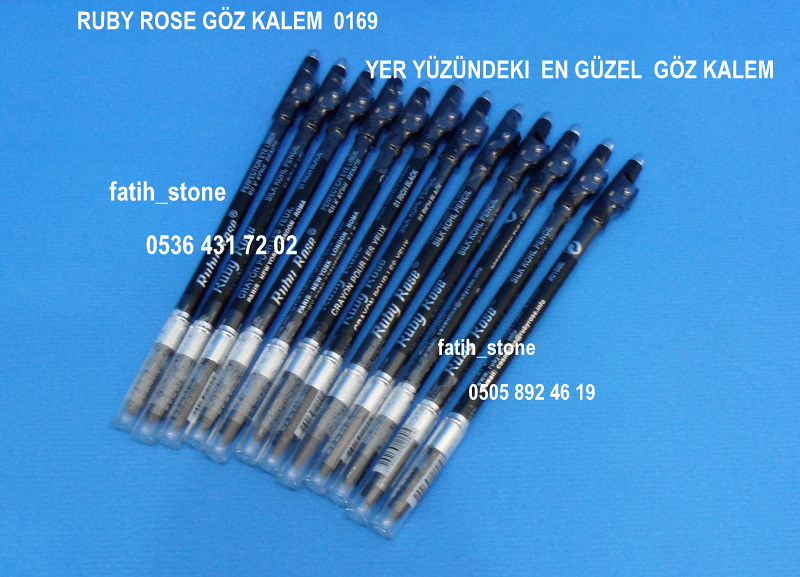The image depicts a collection of 12 to 15 eyeliners arranged closely together on a light blue background. Each eyeliner has a black body with a transition to a silver section and then a gray tip covered by a clear plastic cap. The eyeliners are predominantly labeled "Ruby Rose," with additional inscriptions such as "Silk Coal Pencil," "Rich Black," "Perfection Eyeliner," and "Crayon Pour Les Yeux," confirming they are indeed eyeliners. 

In the top left corner of the photo, there is text that reads "Ruby Rose, GOC, GOZ, Calum, 0169," followed by text in a different language: "YER YUZUNDEKI EN GUZEL GOZKALEM." Along the left side, the text reads "F-A-T-I-H underscore stone" with the number sequence "0536 431 72 02." This text is repeated in the bottom right of the image with the number "0505 892 46 19."